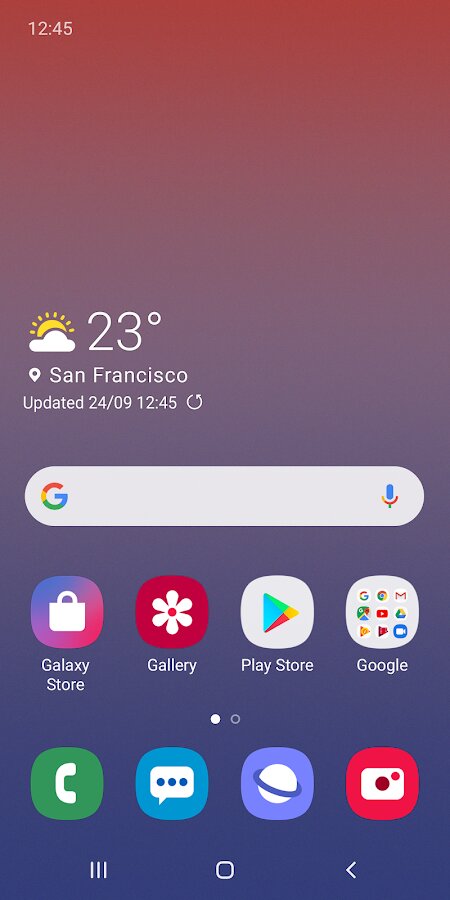Screenshot of an Android Phone Home Screen:

The home screen features a captivating ombre background that transitions seamlessly from a darkish red, maroon at the top, to a deep purple at the bottom. At the top left corner, the time is displayed in white as "12:45." Below this, on the middle left of the screen, there's a weather icon showing a sun partially obscured by a cloud, accompanied by a temperature reading of "23 degrees" in white to its right.

Underneath the weather information, a location icon followed by the text "San Francisco" is visible, also in white. Continuing down, there is a timestamp reading "updated 24/09, 12:45" with a refresh button adjacent to it. Below this section, a prominent Google search bar spans the width of the screen, featuring the colored "G" icon on the left and a colored microphone icon on the right.

The home screen also displays a row of app icons with corresponding labels beneath them. From left to right, these are:
1. Galaxy Store - represented by a white shopping bag icon
2. Gallery - represented by a white flower on a red background icon
3. Play Store - represented by a colored play button on a white background icon
4. Google - represented by a composite icon showing multiple Google apps

At the bottom of the screen, there are four essential functional icons:
1. Phone (represented by a phone receiver icon)
2. Messaging (represented by a chat box icon)
3. Internet/Browser (represented by a planet icon)
4. Camera (represented by a camera icon) 

These icons provide quick access to fundamental phone functionalities. The clean layout and rich background harmonize to provide both aesthetic appeal and practicality.